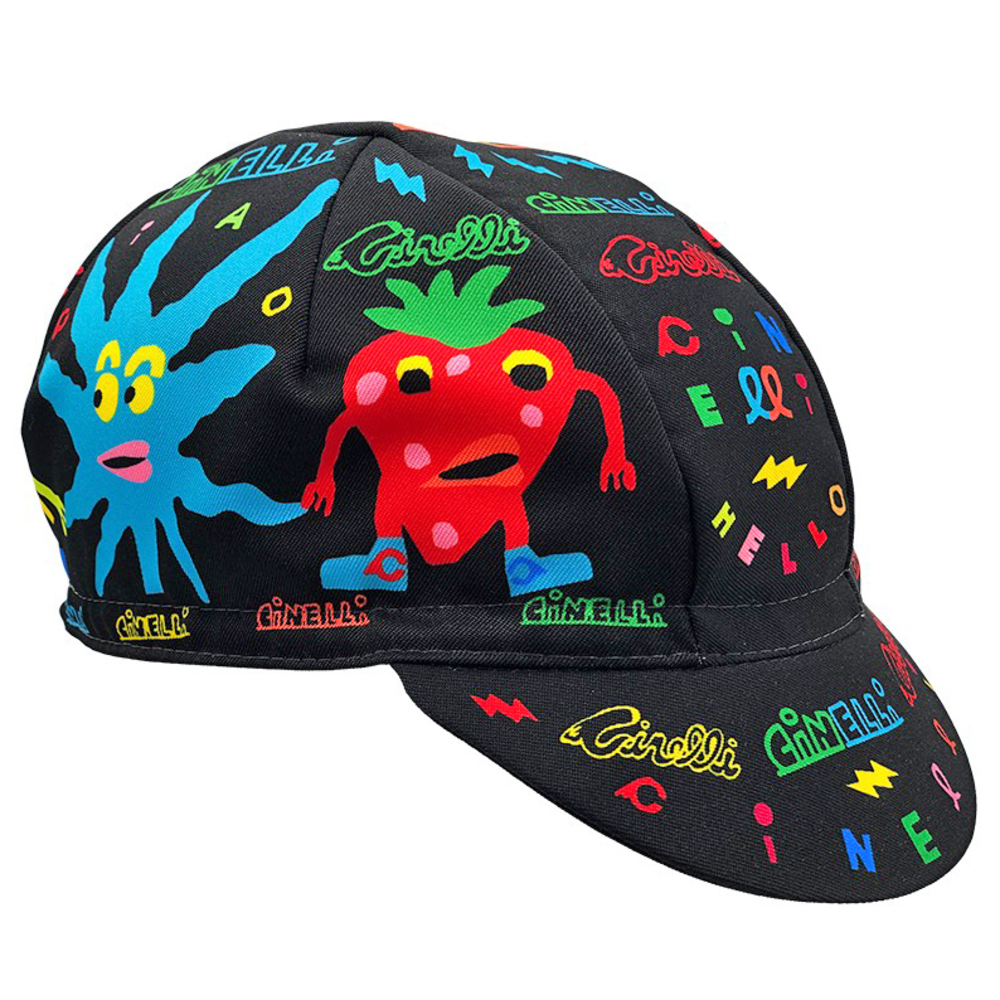The image displays a black hat with a short, train conductor-style bill that is richly adorned with colorful designs and writing. Prominently featured on the hat is a red strawberry character with yellow and black eyes, a green stem, blue tennis shoes, and pink dots. The strawberry has black eyes on a yellow background and pink lips, with its arms hanging by its sides. Alongside the strawberry is a blue starfish-like creature with multiple appendages, yellow eyes, and pink lips. One of the starfish's arms appears to be holding hands with the strawberry. The hat is covered in vibrant details, including lightning bolts in blue and yellow, and recurring words such as "CINELLI" and "hello" in various colors. The lively and intricate patterns suggest the hat might appeal to children, but its sophisticated design could make it suitable for adults as well.